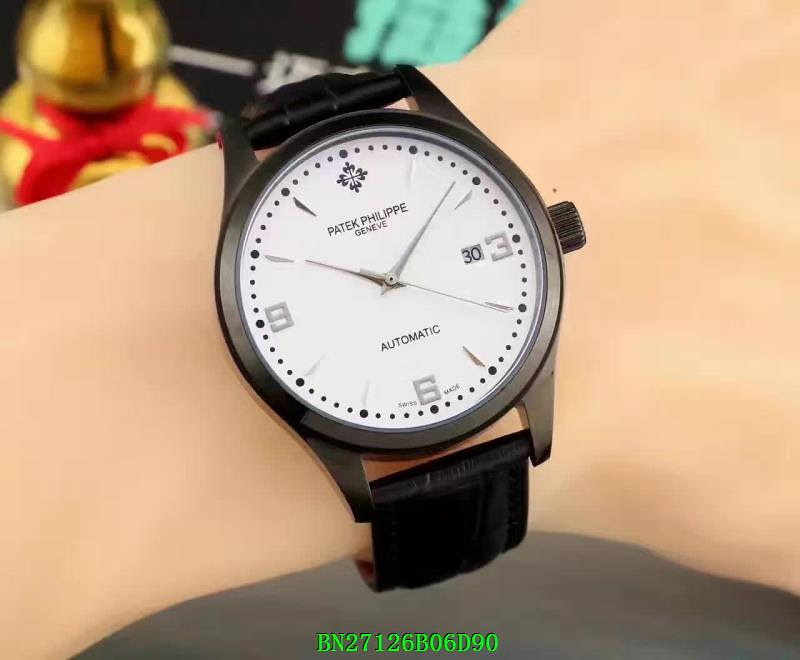This image depicts a detailed close-up of a Patek Philippe wristwatch, seemingly worn on a digitally-rendered wrist. The watch, crafted in Genève, Switzerland, features a white dial face displaying the brand name "Patek Philippe" and the word "Automatic" at the bottom. The face is adorned with black and silver details, including a distinctive design at the 12 o'clock position resembling a combination of swords or a stylized four-leaf clover. Only three numerical markers—3, 6, and 9—are present, rendered in light gray. At the 3 o'clock position, a black date indicator displays the number 30. Surrounding the dial are black circles marking every five minutes, with smaller circles representing the minutes in between. 

The watch's outer casing is smooth, black, and likely metallic, while the band is also black. Interestingly, the wrist appears almost mannequin-like, contributing to the overall digital or 3D model aesthetic. In the image background, there is a golden ornament with a red ribbon, adding a decorative yet unrelated element to the composition. Additionally, green letters "BN27126B060" appear at the bottom of the image, hinting at a potential model number or serial code. Overall, the watch points to 10:09, captured from the perspective of the wearer.